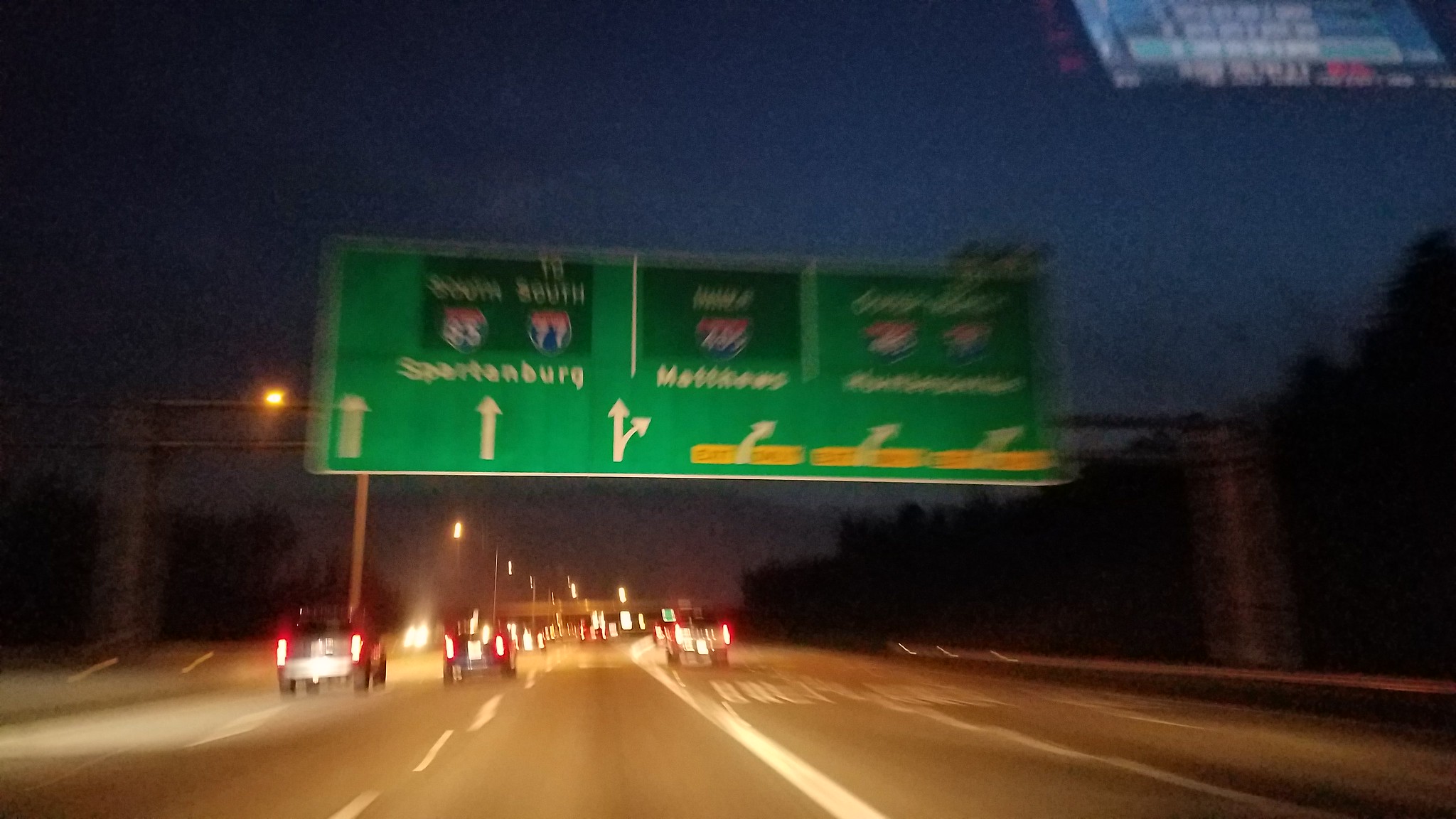The image depicts a nighttime view of an American interstate highway taken from inside a vehicle, likely through a dash cam. The scene is illuminated by streetlights and the blurry glow of taillights ahead. A large green overhead sign spans the highway, suspended on steel beams. This sign directs traffic to "Spartanburg" for three lanes and another destination, possibly "Metzerthau," for the remaining lanes, although the latter is too blurry to read clearly. The sign also includes interstate route numbers, likely I-85 and I-77. There are five visible lanes of traffic, with a solid white divider just to the right of the vehicle. The driver is in the third lane from the left, which appears to be one of the straight-ahead lanes. Trees line the sides of the highway, silhouetted against the dark evening sky.